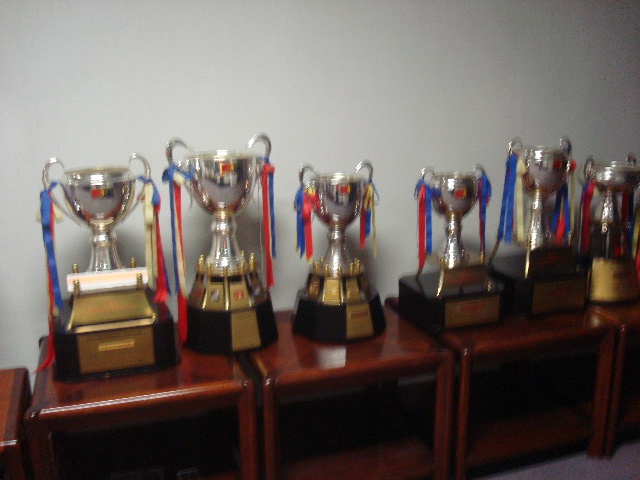This slightly out-of-focus photograph captures six large cup-style trophies arranged in a line on top of five identical, glossy cherry side tables lined up against a white wall. Each trophy, varying in size and base shape—ranging from round to square and trapezoidal—features two handles adorned with hanging ribbons in red, blue, and yellow. The brass nameplates on the trophies are not legible due to the blurriness of the image. The image is taken at a slight angle, about 30 degrees to the left, making the alignment of the trophies appear to slope away from the viewer. The side tables are low to the ground, approximately two feet tall, and the room has a light gray, low-pile carpet. The photograph is lit from the left.